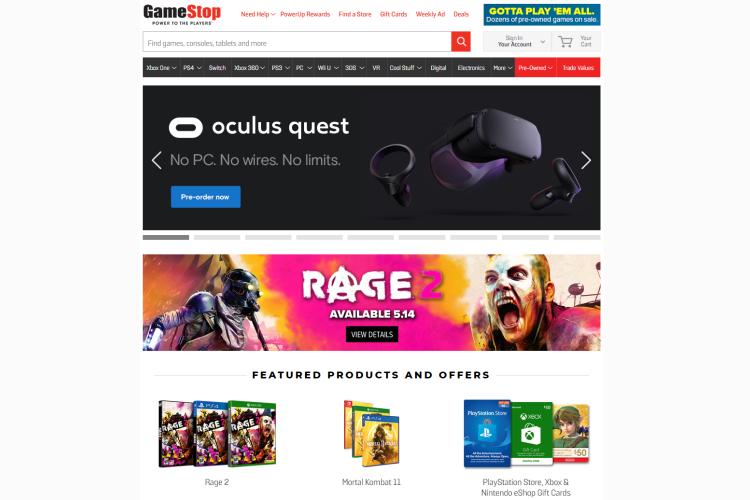The GameStop website features a plethora of information and vibrant visuals designed to attract avid gamers. In the top left corner, the iconic GameStop logo features the word "Game" in black and "Stop" in bold red. Below the logo, in smaller black letters, the slogan "Power to the Players" is prominently displayed.

From left to right, the site's primary navigation bar includes links in red for "Need Help," "PowerUp Rewards," "Find a Store," "Gift Cards," "Weekly Ad," and "Deals." Underneath this navigation bar is a banner with a search field inviting users to "Find games, consoles, tablets, and more" accompanied by a red search button with a white search icon.

On the right side of the header, options to "Sign In" to an account and view the shopping cart, labeled "Your Cart," are available. 

A black navigation bar beneath this header lists several categories in white text, including "Xbox," "PS4," "Switch," "Xbox 360," "PS3," "PC," "Wii U," "3DS," "VR," "Collectibles," "Digital," "Electronics," and "More." 

Below this, two red banners feature options for "Pre-Owned" and "Trade Values." A prominent black section with an "Oculus Quest" advertisement boasts "No PC, No Wires, No Limits," with a "Pre-Order Now" button in a blue banner with white text. The ad includes an image of the device in black, with an arrow for scrolling to view additional photos.

Subsequent to the Oculus Quest section, an advertisement for "Rage 2" stands out. The word "Rage" is in white, with the numeral "2" in pink, accompanied by a release date of "Available 5-14." The background features an intense pink and yellow design with a screaming man on the right and an alien-like figure on the left. A black "View Details" banner is also visible.

Further down, a "Featured Products and Offers" section displays three main categories. The "Rage 2" category shows three game thumbnails. In the middle, "Mortal Kombat 11," also showcases three games. On the right, the "PlayStation Store," "Xbox," and "Nintendo eShop" gift cards are presented, with three gift cards displayed under each respective category.